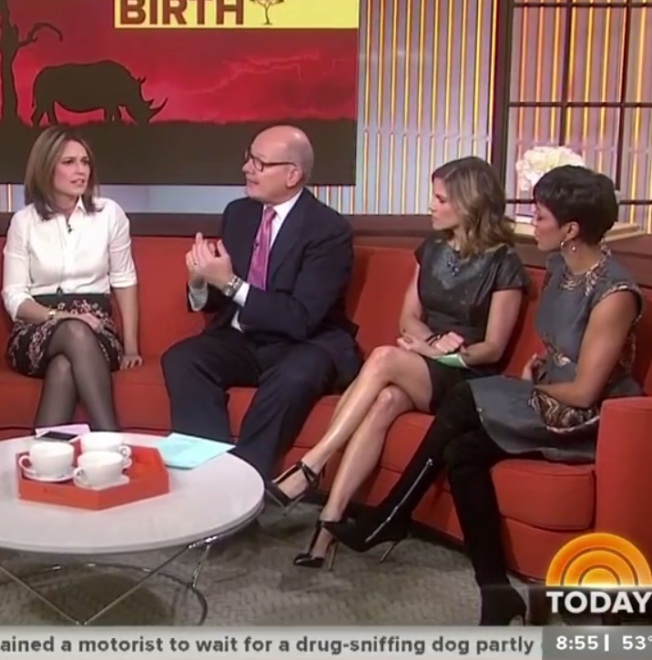This image is a screenshot from a live episode of the Today Show, featuring a talk segment. The backdrop includes a nature-themed poster with a striking red sky and black ground, depicting a rhino, and the word "birth." The screen displays the caption "Today" along with a subtext about motorists waiting for a drug-sniffing dog, indicating the time as 8:55 a.m. and a temperature of 53 degrees.

The scene is set in an indoor studio with a large, curved red couch where four individuals are seated. Starting from the left, a woman with shoulder-length brown hair is wearing a white blouse paired with a black and colorful flower-patterned skirt and black pantyhose. Next to her, a bald man with glasses dressed in a black suit, white shirt, and purple tie, adorned with a gray wristwatch and a wedding band on his left hand, is engaging in conversation with her. To his left sits another white woman with shoulder-length wavy brown hair, dressed in a black dress and black shoes. At the far right, a light-skinned black woman with very short black hair, wearing hoop earrings, a gray dress, black stockings, and black high-heel boots, completes the lineup. In front of them is a white coffee table with three white coffee cups on red plates and a blue piece of paper. The floor is carpeted in gray, tying the scene together.